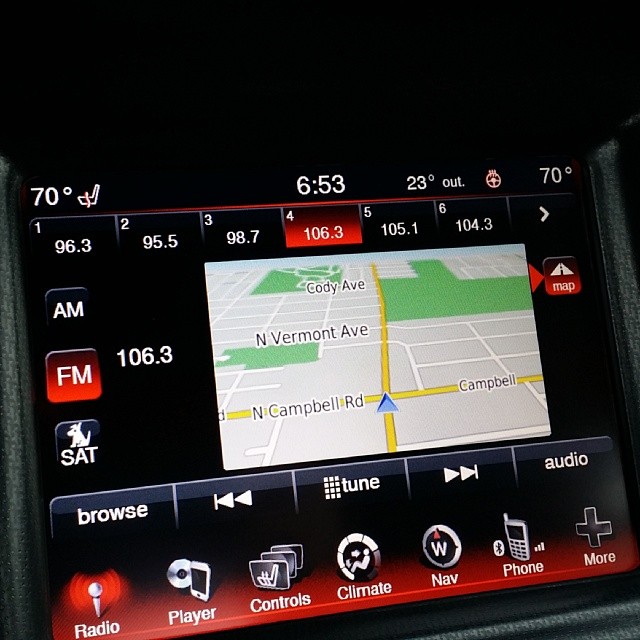The image depicts a GPS screen set against a black background, likely viewed from inside a car's dashboard. The primary focus is a gray GPS display marked with yellow lines and labeled road names, including Cody Avenue, North Vermont Avenue, and Campbell Road. The map indicates the car is about to cross North Campbell Avenue, heading towards North Vermont Avenue and Cody Avenue. Surrounding the GPS screen are various controls and information. The top section shows preset radio stations, with the current station being 106.3 FM on channel 4. The climate controls show the internal temperature set to 70 degrees Fahrenheit (23 degrees Celsius outside). The time displayed is 6:53, and additional options include controlling the radio, CD player, phone connectivity, and climate settings. The dashboard combines navigation, entertainment, and climate control functionalities into a single integrated system.